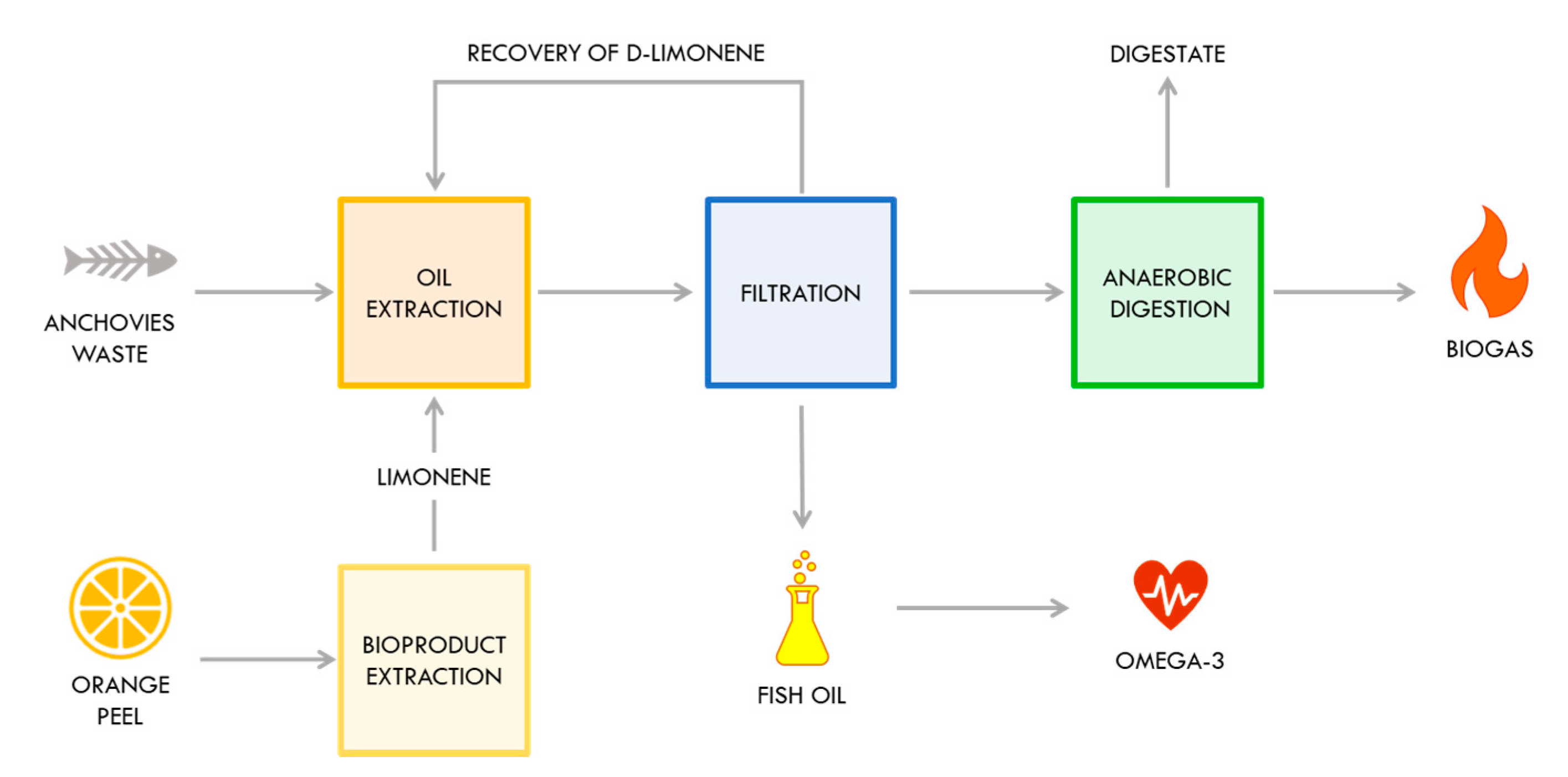This intricate diagram illustrates the interconnected extraction processes of bioproducts from anchovies waste and orange peels against a white background. The process begins in the upper left corner with an icon of a gray fish skeleton labeled "anchovies waste." A gray arrow points to an orange-bordered box labeled "oil extraction." Another gray arrow leads to a blue-bordered box labeled "filtration." From "filtration," there's a gray arrow pointing to a green-bordered box labeled "anaerobic digestion," which has an upward gray arrow to the label "digestate" in the upper right corner. To the right of "anaerobic digestion," another gray arrow points to a "biogas" label represented by an orange flame icon.

On the lower left corner, the process begins with an icon of an orange slice labeled "orange peel," leading via a gray arrow to a yellow-bordered box labeled "bioproduct extraction." This box connects upward to the "oil extraction" box via a gray arrow. Additionally, "filtration" connects back to "oil extraction" through several gray lines labeled "recovery of d-limonene." 

Below "filtration," a downward gray arrow points to a flask icon labeled "fish oil," which is also connected by a gray arrow to the label "omega-3," represented by a heart icon with white line patterns in the lower right corner.

All text within the diagram is in capital letters and utilizes color-coded borders—yellow, orange, blue, green, and gray—with lighter shades inside the boxes.